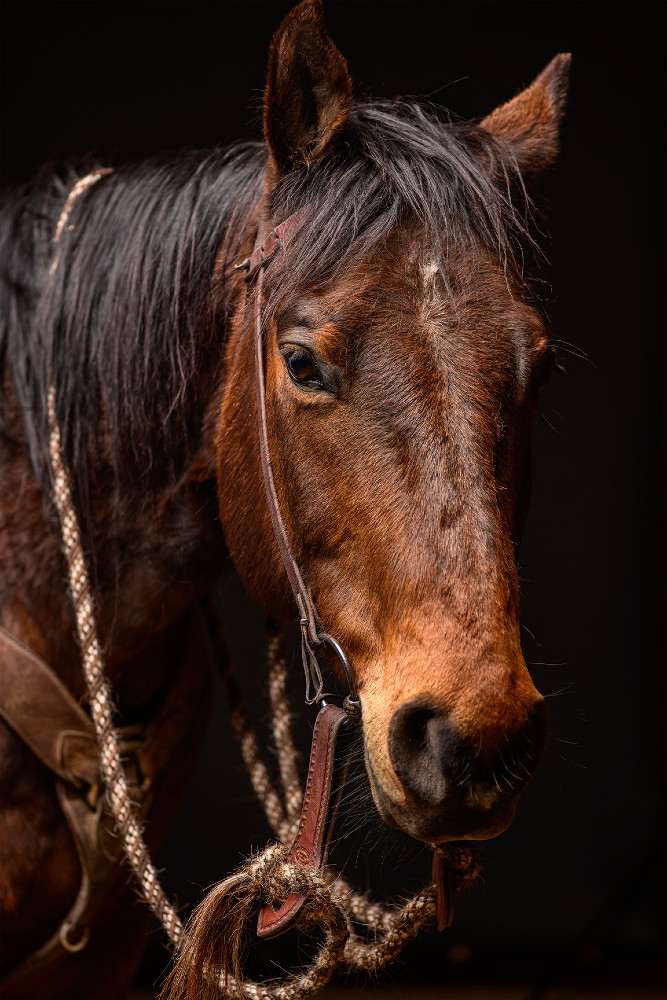This striking portrait-style photograph captures the head and upper chest of a dark brown chestnut-colored horse with a glossy black mane, set against a deep black background. The horse, wearing a leather bridle with a bit in its mouth, has black eyes that gaze forward, giving an intense and captivating look. The bridle’s reins are crafted from a distinctive brown and white braided rope, extending from the bit where the rider would steer the horse. The horse’s fur is a rich, dark brown that becomes slightly lighter towards the end of its nose, contrasting beautifully with the dark fur along its jaw and the black mane. Illuminated by light, the horse's coat gleams, enhancing the texture and depth of its appearance. The small, furry brown ears blend seamlessly into the dark mane, adding to the horse’s noble and handsome demeanor.